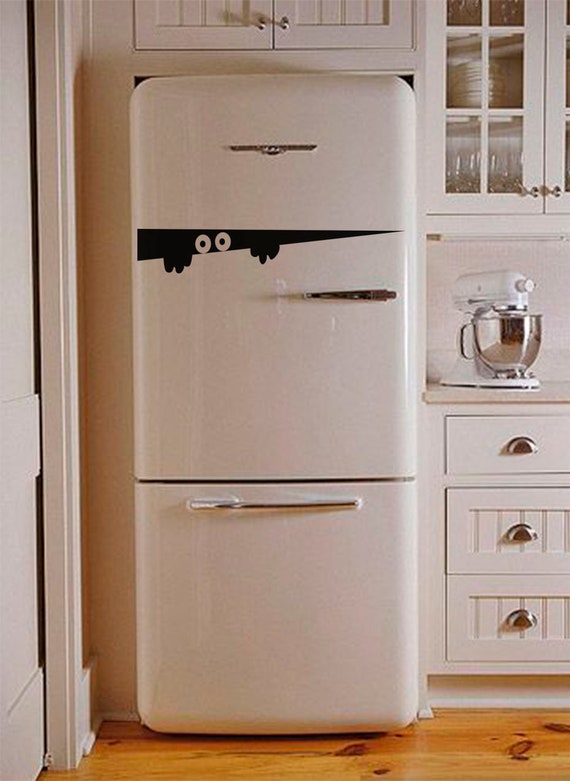The photograph showcases a well-lit kitchen centered around a tall, white, old-style refrigerator with curved edges and a large bottom freezer, complete with a long silver handle. A unique decal adorns the refrigerator's top section, depicting a creature peeking out; this effect is created using a black triangle, white eyeballs shining from the darkness, and small black hands. To the refrigerator's right, a counter holds a large white mixer, with a set of three drawers below and a white cabinet with glass panes above, revealing plates and cups inside. The kitchen wall to the left features a sliding white door, and the shiny wooden floor, with planks running horizontally, adds warmth to the scene. Overall, the image is clear and brightly lit, emphasizing the details of this cozy kitchen setting.